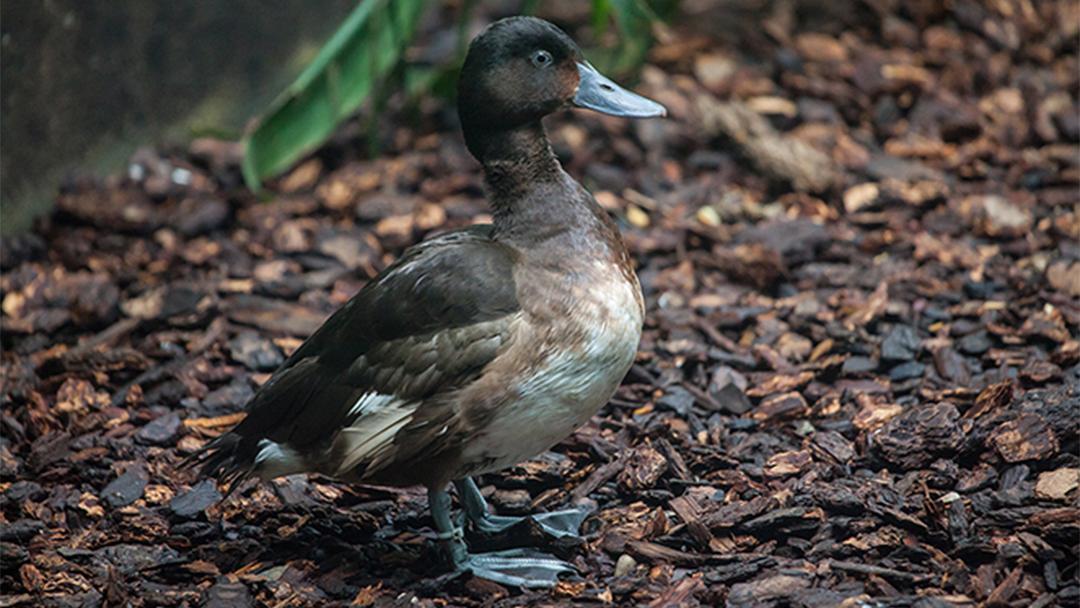In this rectangular image, we see a close-up profile of a duck standing on a bed of brown and black wood chips. The duck is facing right, revealing a dark brown head with a gray iris and a dark pupil. Its bill is slightly curved and gray with a visible black nostril line towards the upper portion. The duck has a moderately long neck, transitioning from dark brown to a lighter gray below, and a distinctive white chest. Its folded wings are primarily black with a tinge of white at the edges. The tail feathers are dark brown and slightly ruffled. The duck stands on webbed gray feet, with a noticeable band around its right leg, which is closest to the viewer. In the background, there is a small plant with leaves hanging down. While there is no visible water, an undefined area in the upper left corner suggests the possible presence of a pond. Overall, the surroundings and the duck's plumage present a contrast between dark, earthy tones and lighter, prominent whites on its chest.